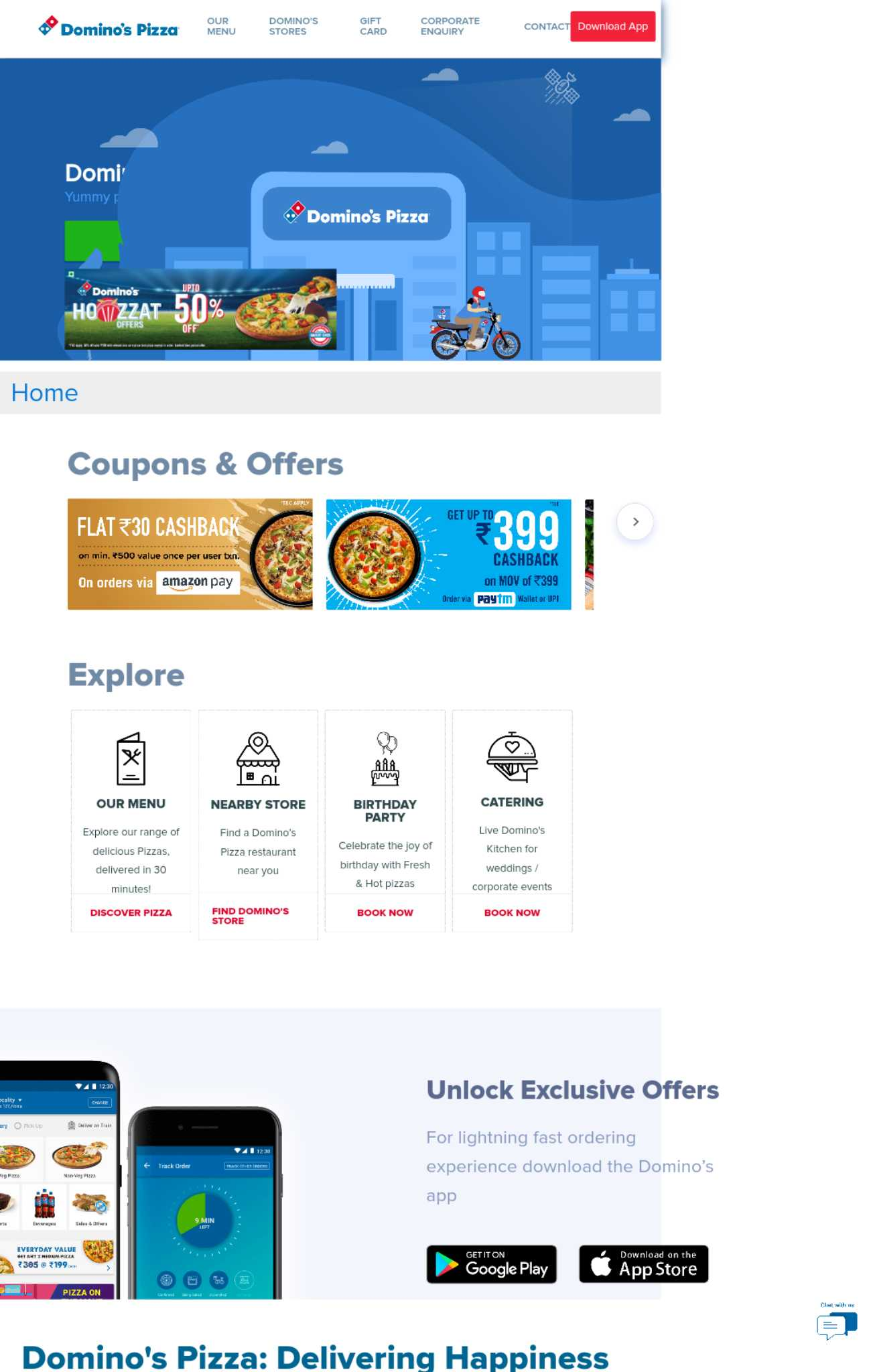The website for Domino's Pizza features a clean white navigation bar at the top, prominently displaying the iconic Domino's logo; the familiar red and blue domino is accompanied by the small text "Domino's". The navigation options available include subsections like "Domino's Stories," "Gift Cards," "Corporate Inquiry," "Contact," and a red button with an unreadable label, in addition to a "Home" button.

Just below the navigation bar, the site is segmented into various sections. One section titled "Coupons and Offers" highlights deals such as "Flat 30% Cashback" and options to "Pay and Own Orders Via Amazon," with additional offers like "Get Up to $3.99 Cashback," all amid images of delicious pizzas. 

Further down, the site invites users to "Explore" by presenting various options: 
- "Our Menu" for discovering a variety of pizzas
- "Nearby Store" for locating the nearest Domino's outlet
- "Birthday Party" and "Catering" services, each with a "Book Now" option in red.

The lower section of the page showcases images of people engaging with Domino's via their phones, accompanied by the message "Unlock Exclusive Orders." The website wraps up with the motto, "Domino's Pizza: Delivering Happiness."